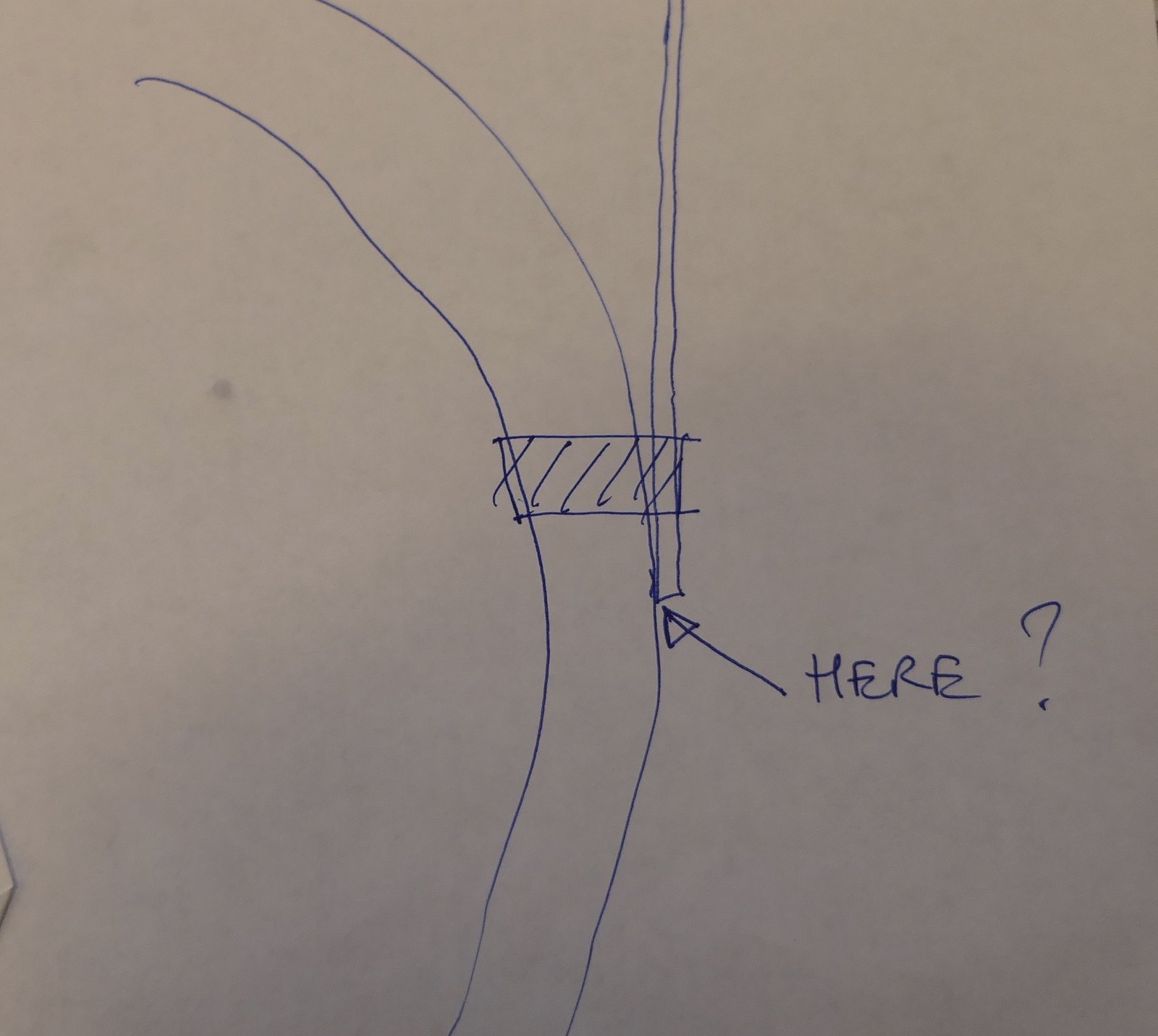In this photograph, we see a close-up image of a hand-drawn map on a piece of paper. The map appears to depict a roadway leading upwards, with an overpass or bridge represented as a rectangle intersected by diagonal lines. An arrow, sketched with a straight line and a triangle at the top, points to an area on the map labeled in capital blue ink letters as "HERE?" The writing and all illustrations are done in blue ink. The paper bears some indications of dirt marks or possibly grains from the camera lens, adding to its slightly grainy texture. The image does not provide any specific context or location details, focusing solely on this rudimentary map and its key elements.